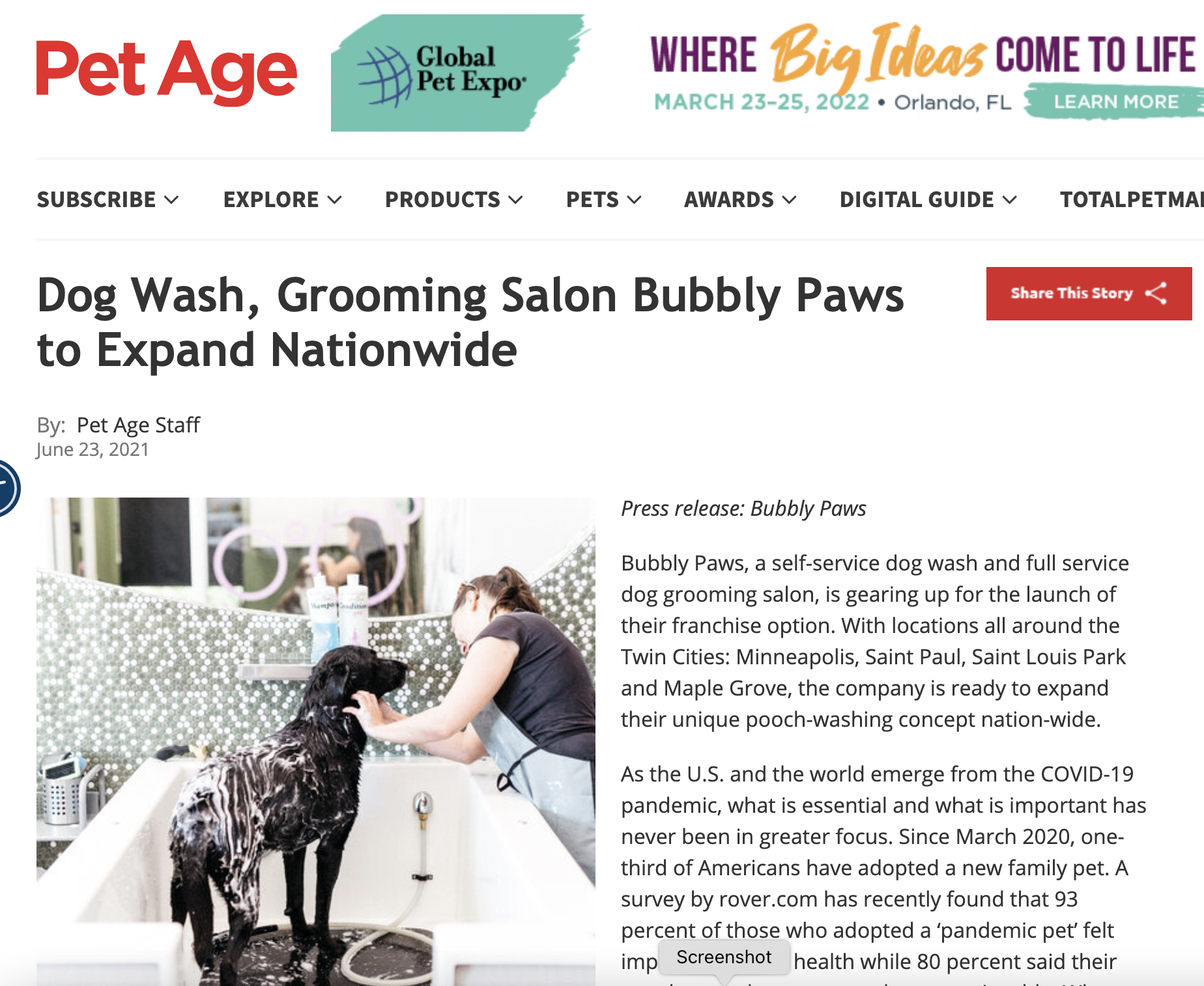The image depicts a screenshot from a website, framed in what appears to be a square-shaped layout with no defined borders. The background is predominantly white, with black font complemented by various colors. 

At the top, a thin gray line creates a header section. Positioned on the top left, the words "Pet Age" are displayed in red, followed by a paint stroke-like image labeled "Global Pet Expo." This image features a grid-patterned globe to its left; the background is green, the globe is blue, and the text is in black. To the right of this logo, the phrase "Where Big Ideas Come to Life" is presented, with "Where" and "Come to Life" in purple, and "Big Ideas" in orange. Below this, the dates "March 23rd to 25th, 2022 in Orlando, Florida" are listed in green, accompanied by a green link encouraging users to learn more.

Further down, there are several drop-down menus delineated by thin gray lines on the top and bottom. These menus are labeled as "Subscribe," "Explore," "Products," "Pets," "Awards," "Digital Guide," and "Total Pet Something," although the last label is cut off.

Beneath these menus, a headline reads "Dog Wash Grooming Salon Bubbly Paws to Expand Nationwide," followed by a photograph of a woman washing a dog that appears to be a black labrador. Beneath this image, the label "Press Release" appears alongside the name "Bubbly Paws," leading into a two-paragraph article. 

At the top right corner, a red box with white font offers the option to "Share This Story."